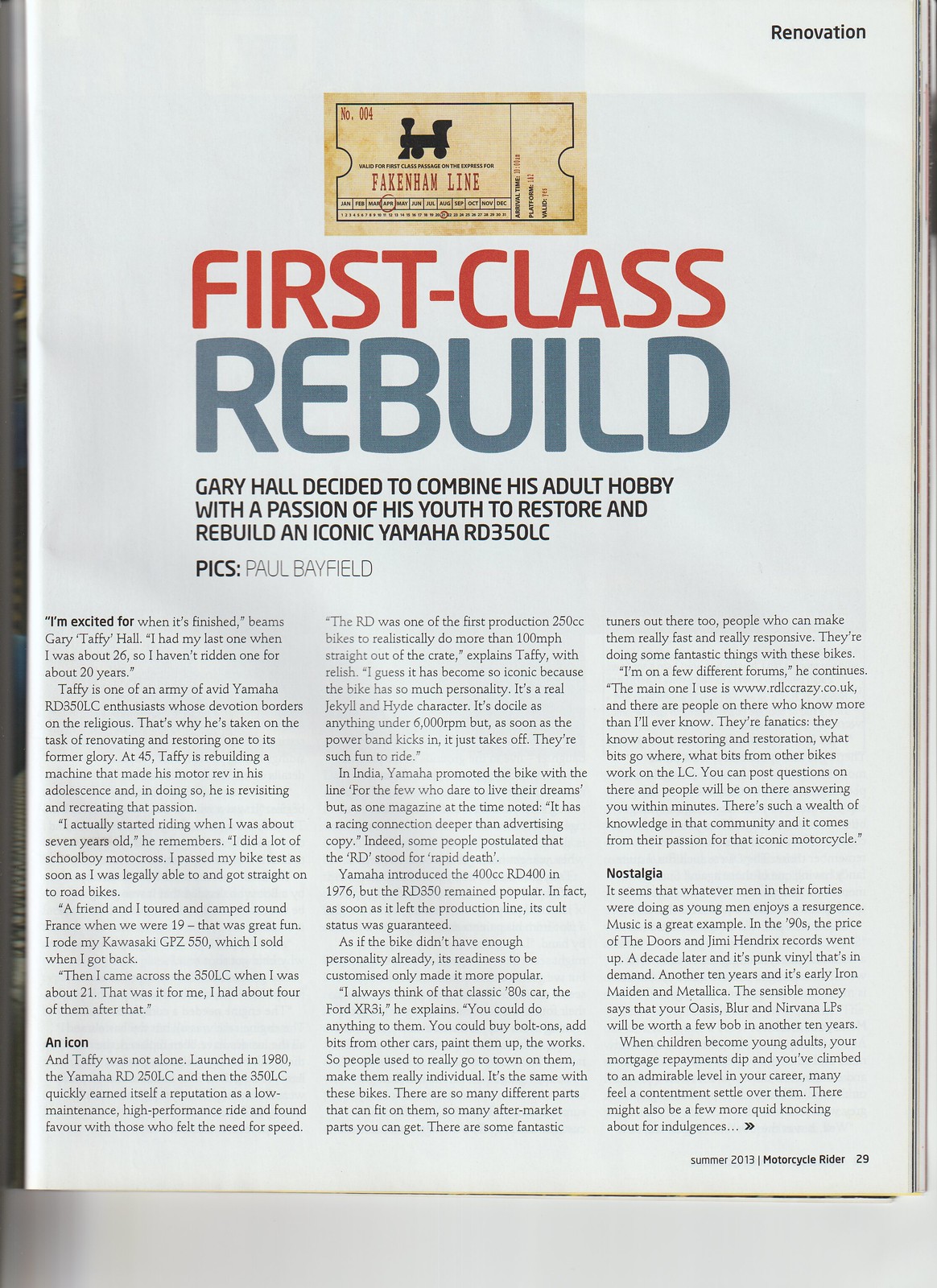This image shows a magazine cutout placed within a frame, featuring an article about a classic motorcycle renovation. The top left and right corners bear the headline "Renovation." Central to the image is a train ticket motif, with a serial number "004" on the top left and a black train engine logo beneath it. The ticket also reads "Valid for first class passage on the express for Feckenham line," in bold red letters. Below this, a calendar displays all twelve months in individual boxes, with April circled in red ink. Similarly, the date "21" is circled within the days numbered 1 to 31. On the right of the ticket, details such as "Arrival time: 10.00 a.m.," "Platform: 1 and 2," and "Valid: Yes" are listed.

Directly below the ticket image, the headline "First Class Rebuild" is prominently displayed, with "First Class" in red and "Rebuild" in gray. The subheading elaborates: "Gary Hale decided to combine his adult hobby with the passion of his youth to restore and rebuild an iconic Yamaha RD 350 LC." The article, authored by Paul Bayfield, features an interview within quotations: "I'm excited for when it's finished," says Gary "Teffy" Hall. Teffy shares that his last experience with the motorcycle was two decades ago when he was 26. Now, at 45, he is ardently working on refurbishing the Yamaha RD 350 LC, a motorcycle that left an indelible mark on his youth.

The article details Teffy's journey with motorcycles, starting from his early years: "I started riding when I was about seven," he recalls. He narrates his history with various bikes, emphasizing the significance of the Yamaha RD 350 LC, which he encountered at 21 and owned multiple times thereafter. The piece underscores the motorcycle's historic impact, highlighting its low maintenance and high performance, which made it iconic since its launch in 1980.

Teffy marvels at the bike's customizable nature, comparing it to the classic Ford XR3 for its versatility in modifications. He notes the vibrant community of enthusiasts and experts who share their profound knowledge on forums like www.rdlccrazy.co.uk, facilitating restorations and offering advice.

The article concludes with a reflection on nostalgia, likening the resurgence of classic motorcycles among men in their 40s to the rekindling of interest in vintage music records over the decades. The bottom right corner of the cutout indicates the source: "Summer 2013 Motorcycle Rider, page 29."